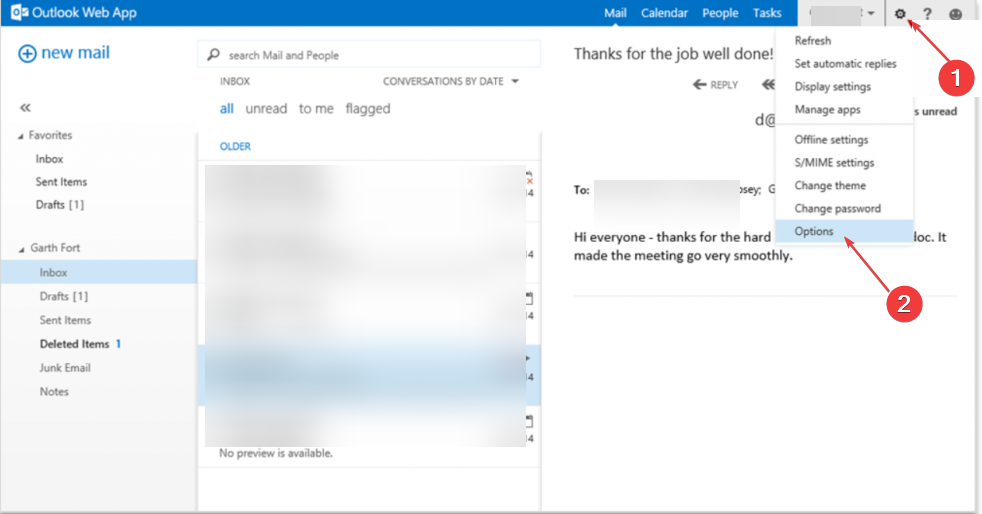The screenshot depicts the Outlook Web App interface with a prominent blue navigation bar at the top. On the left side of this bar is the Outlook Web App logo. The top right corner features navigational tabs for Mail, Calendar, People, and Tasks. Additionally, a gear icon dropdown menu is visible, indicating a selection of settings.

There is a bright red circle marked with a '1' and an arrow pointing towards the gear icon. This indicates that the gear icon has been clicked to display the dropdown menu. The dropdown options from the gear icon include: Refresh, Set Automatic Replies, Display Settings, Manage Apps, Offline Settings, S/MIME Settings, Change Theme, Change Password, and Options. The 'Options' item is highlighted in a light blue color, drawing attention to it. Another red circle marked with a '2' and an arrow points specifically to this highlighted 'Options' entry.

In the central section of the screen, an email is partially visible. The email list pane to the left of the selected email is blurred for privacy, obscuring any details of other emails. The visible email content shows a greeting, "Hi everyone," followed by partial text, "thanks for the hard blah, blah, blah. It made the meeting go very smoothly," with the remainder of the email cut off.

On the far left side of the screen is a navigation panel with options to compose a new email and access various email folder sections. These include Favorites, Inbox, Drafts, Sent Items, Deleted Items, Junk Email, and Notes.

This detailed view of the Outlook Web App provides insight into the app's user interface, layout, and available options for managing emails and account settings.